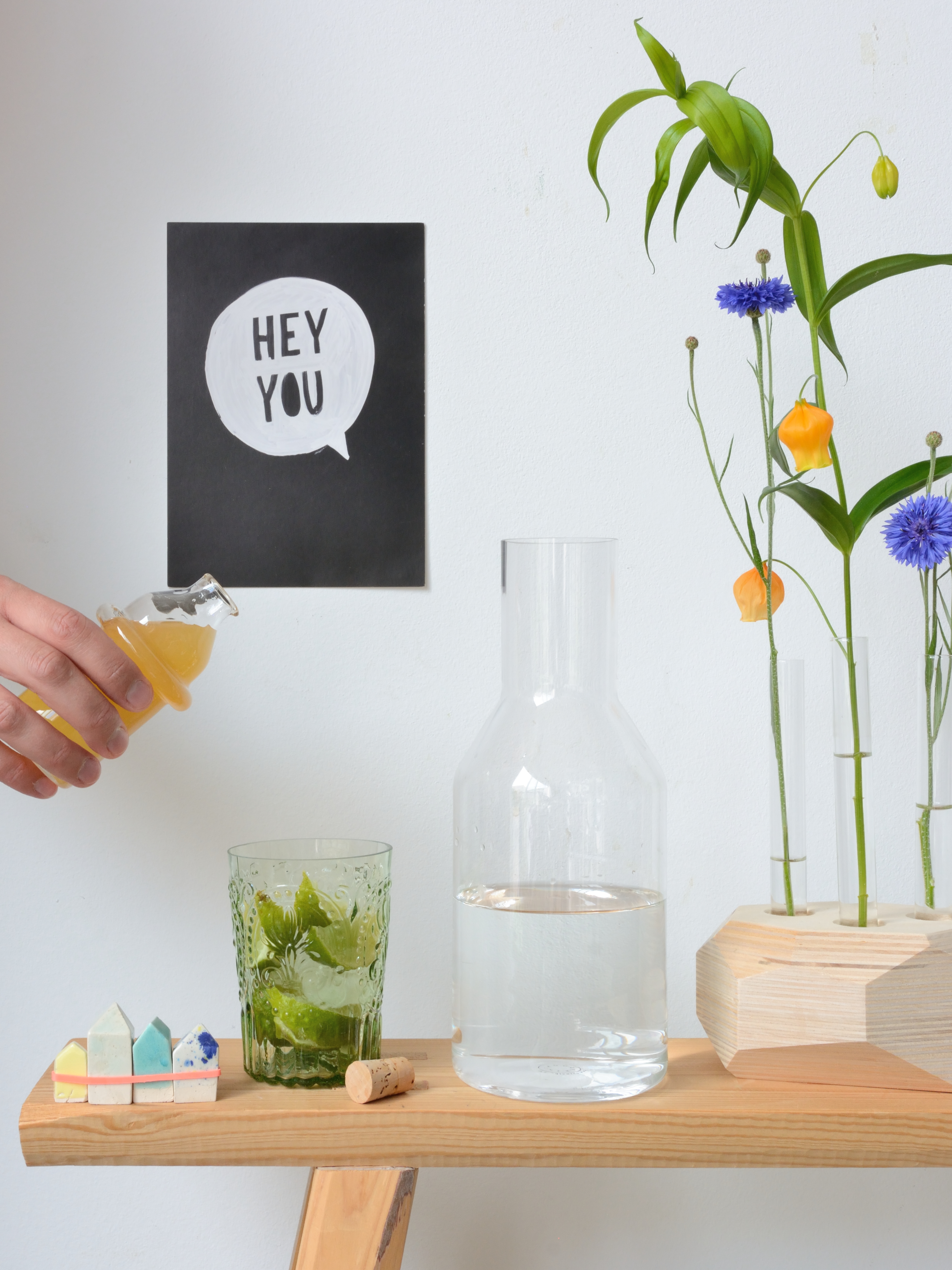This photograph features a meticulously arranged still life composition. On the left side of the image, a hand delicately holds a glass jar of orange juice, poised high above a decorative glass that contains fresh lime slices. Though the jar is lifted, the juice has yet to be poured. The glass itself is ornate, featuring an intricate, raised design.

To the left of this glass, there's a set of four small, colorful pyramid-shaped objects that resemble soaps. These miniature pyramids, varying in height from about an inch to an inch and a half, are bundled together with a pink rubber band. The colors include yellow, white, light blue, and another white one with dark blue spots.

In front of the glass sits a solitary cork. All these items rest on a piece of unfinished wood, likely part of a table, revealing only one visible table leg. The wood exudes a warm, maple hue.

To the right of the decorated glass is a large water pitcher. The round base of the pitcher narrows into a long neck, currently filled with water. Further to the right, a wooden pot holds three glass test tubes, each showcasing a different flower. The two outside test tubes contain blue flowers resembling asters, whereas the middle test tube holds two orange, lantern-shaped blooms with long leaves.

In the background, affixed to the wall, is a black piece of paper, probably measuring around 8.5 by 11 inches or slightly larger at 11 by 14 inches. It features a white speech bubble with the words "HEY YOU" written in capital letters, and the center of the "O" is filled in black.

This eclectic mix of items comes together to create a visually captivating and detailed still life scene.